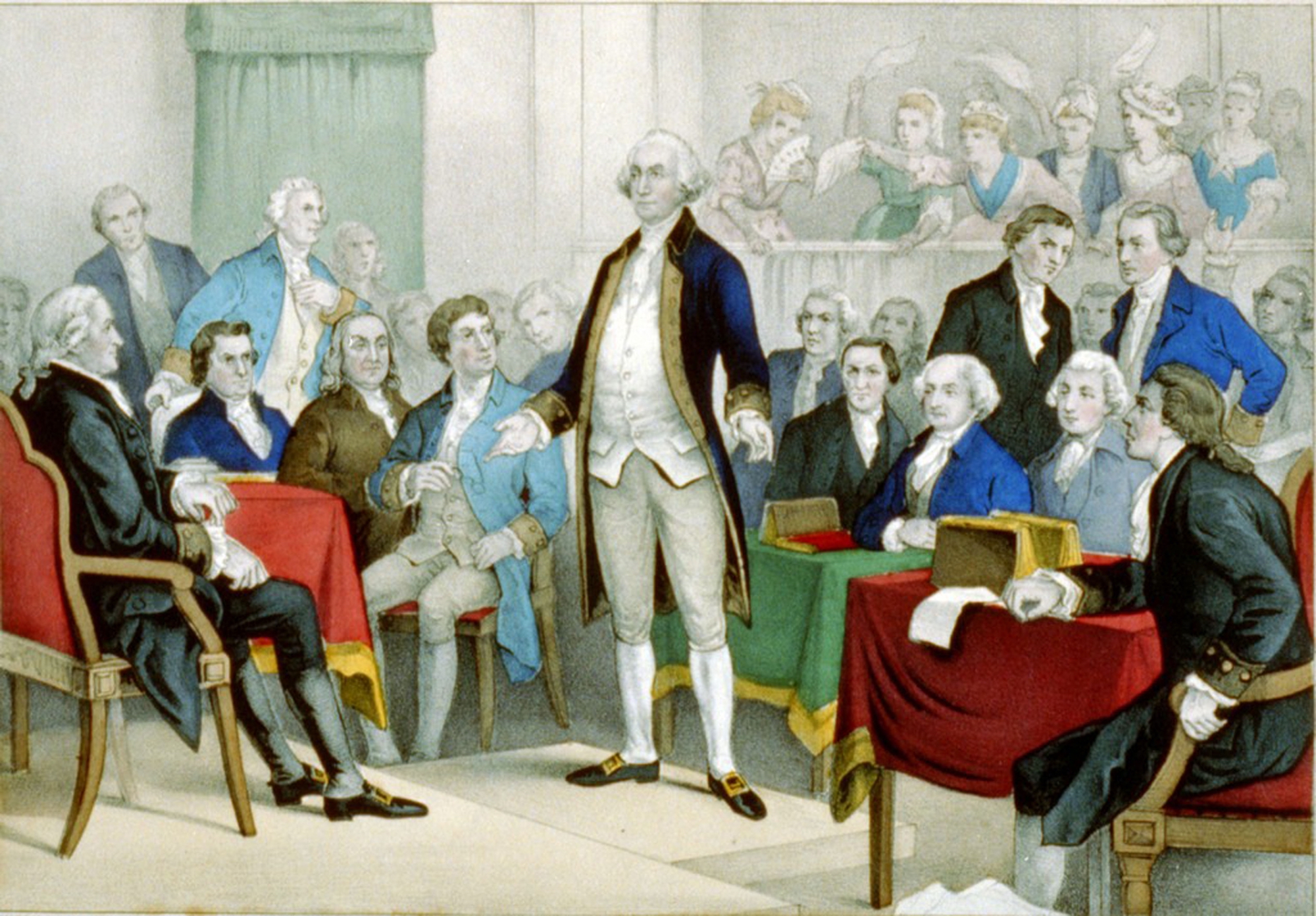The image is a detailed drawing depicting early American history, focusing on a pivotal moment involving the Founding Fathers. At the center stands George Washington, a commanding figure with arms outstretched as if challenging those around him. He is dressed in a long blue coat adorned with gold accents, an unbuttoned white vest, gray pants, white knee socks, and black shoes with gold buckles. His face is characterized by a white powdered wig, pale skin, and rosy cheeks.

Washington is surrounded by a circle of men seated at tables draped with vibrantly colored tablecloths, which include two red ones and one green, each featuring a gold strip along the bottom edge. Among the seated men, Benjamin Franklin can be identified on the left side in a brown coat. To the right, two men appear visibly enraged, having stood up, while two men on the left seem concerned.

In the background, behind a short wall on the right, women are visible in an elevated balcony area. Some are waving handkerchiefs or fans and appear somewhat upset. The setting includes other details such as a white wall and a green curtain over a window, enriching the historical ambiance of the scene.